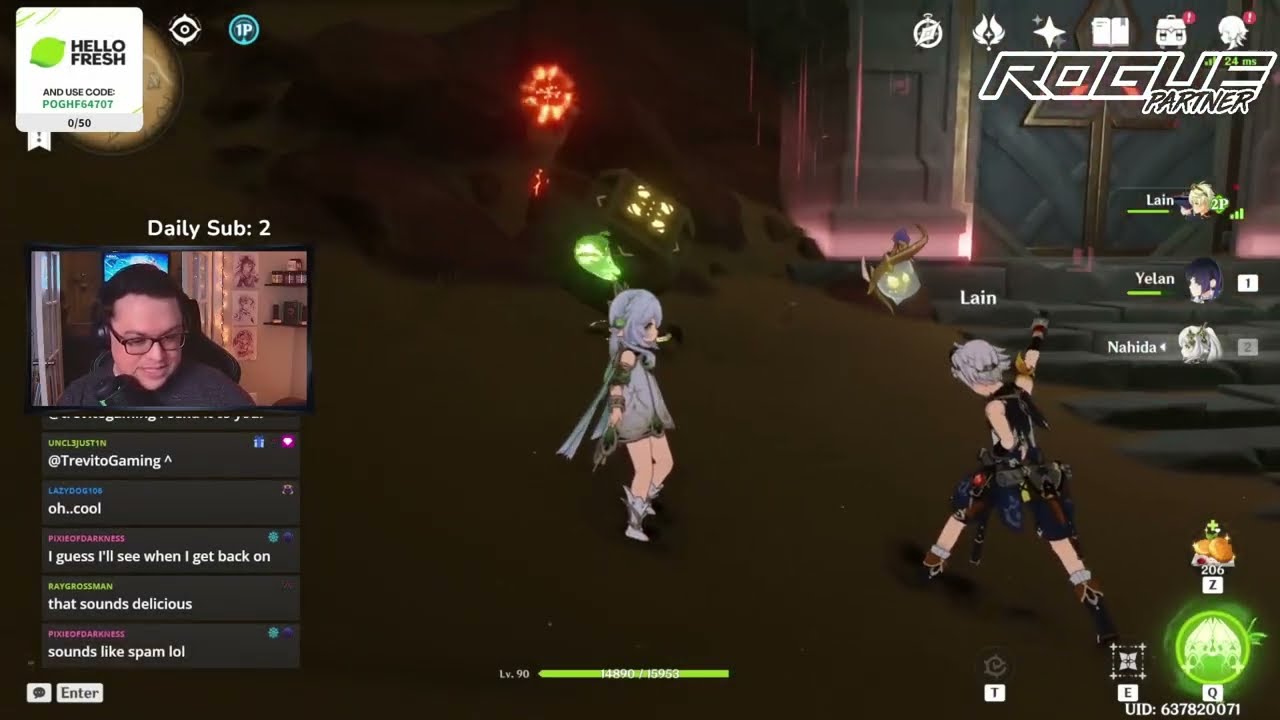The screenshot from a video game features two anime characters standing on a brown-colored ground. The female character, named Lane, has long gray hair and wears a gray dress with a matching cape, holding a hammer as her weapon. The male character, sporting spiky gray hair, is dressed in a black shirt, blue shorts, and black boots, and is pointing towards a metal door on the far right that glows pink on the sides, flanked by pillars. Behind the characters, a building and shining objects are visible.

In the bottom left corner of the screenshot, there is a photograph of the male streamer wearing glasses, a gray shirt, and black headphones, seated in a black gaming chair with a microphone in front of him. This image shows walls and a door in the streamer's room, adorned with pictures. Above the streamer's photograph, chats from viewers are visible, with the text "Daily Sub: 2" prominently displayed.

In the top left corner, a sponsorship logo for "Hello Fresh" appears, along with the text "Use code POGHF64707." In the top right corner, various game-related icons are present, with the text "Rogue Partner" partially transparent. The lower right corner contains game options, adding to the comprehensive gaming interface.